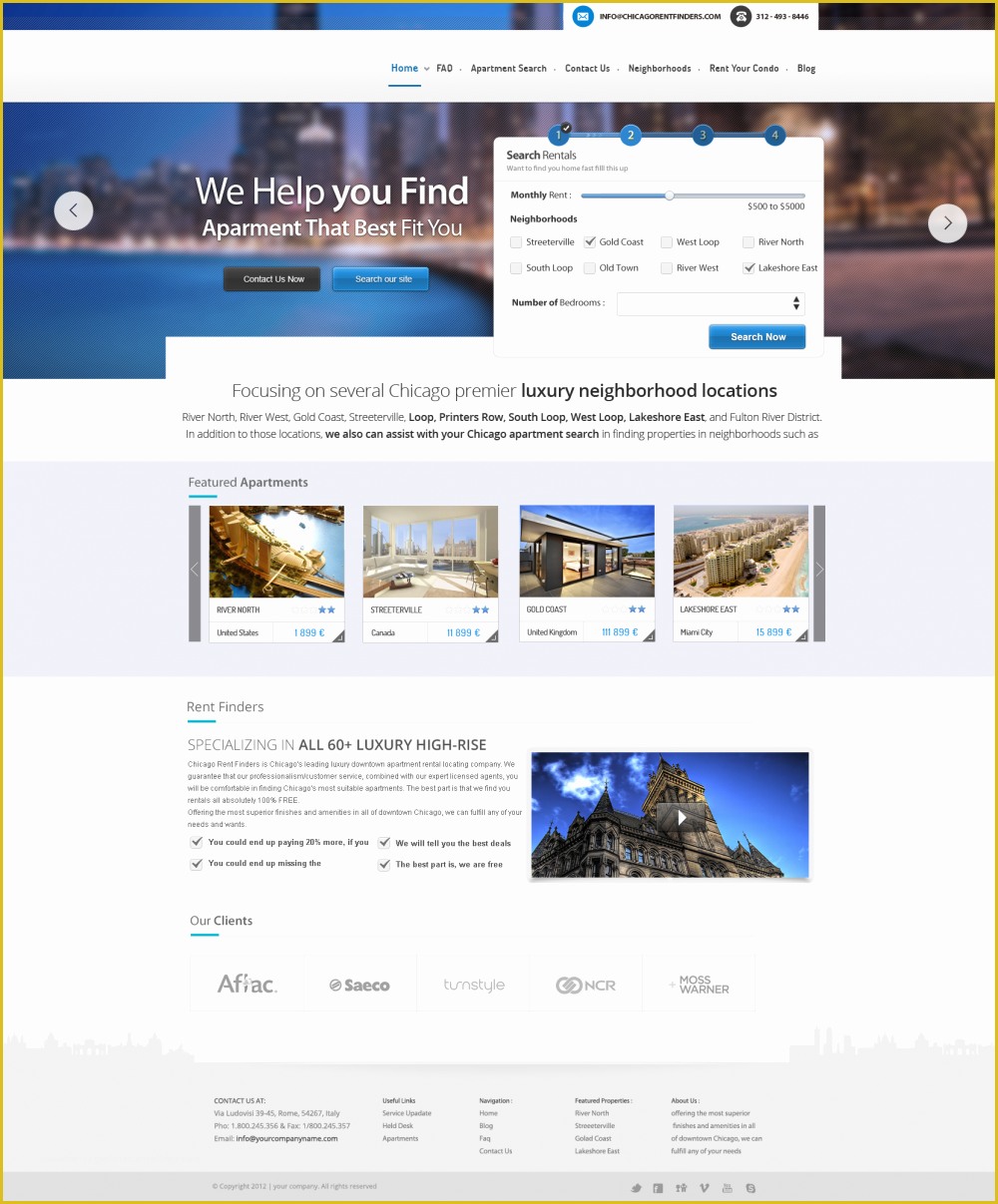In the image, a website interface for "Chicago Rent Finders" is displayed, clearly targeting individuals seeking apartments in Chicago. At the top of the webpage, there's an email address prominently shown as info@ChicagoChicagoChicagoRentFinders.com. Next to it, a phone icon precedes the contact number (312) 493-8446. The navigation bar offers links to various sections including FAQ, Apartment Search, Contact Us, Neighbors, Rent Your Condo, and Blog, with the 'Home' button highlighted in blue.

The background of the webpage features a faded cityscape of Downtown Chicago, giving a bustling urban feel. A bold white text serves as the headline, reading "We Help You Find the Apartment That Best Fits You," with a subheading that reassures users of their service. Below this, a prominent black 'Contact Us Now' button invites user engagement.

The right section of the page displays an interactive white dialogue box labeled 'Search Rentals.' Users can utilize a slider to set their budget range, select desired neighborhoods, and specify the number of bedrooms, followed by clicking a 'Search Now' button.

Additionally, the webpage highlights "Chicago's Premier Luxury Locations" along with ratings and costs of featured apartments. It showcases a list of notable clients including Aflac, Seiko, Turnstile, NCR, and Moss Warner.

At the bottom of the page, there's comprehensive contact information for the company, including their location, phone number, email, and a list of useful links.